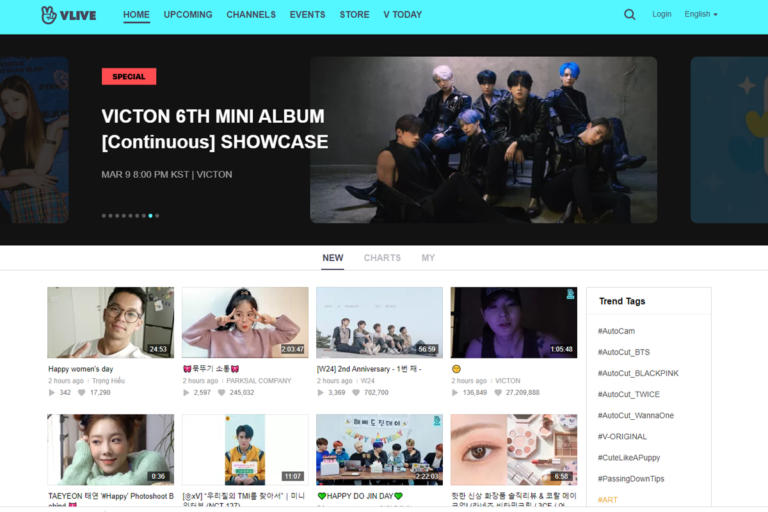This is a detailed screenshot of a web page from the V Live platform, distinguished by a turquoise-colored banner at the top featuring the V Live logo and an icon of a hand making a peace sign. The navigation bar beneath the banner displays several options: "Home" (highlighted), "Upcoming," "Channels," "Events," "Store," "V Today," a magnifying glass icon for "Search," "Login," and "English."

Below the navigation bar is a prominent photograph of a K-pop boy band, presumably VICTON. The members are strikingly handsome, with diverse hair colors including pink, blue, and black. Accompanying the photograph is a caption reading, "Special VICTON VICTON 6 Mini Album Continuous Showcase. March 9, 8 p.m. KST, VICTON."

Further down is a section providing additional options such as "New," "Charts," and "My," followed by an array of video thumbnails labeling various events and topics. These thumbnails include titles such as "Happy Women's Day," a video in Korean script, "W24 2nd Anniversary," a video indicated by a yellow emoji, "Taeyeon, Happy Photoshoot B," another Korean script labeled video, "Happy Dojin Day," and a makeup tutorial, also in Korean.

On the right side of the page, a list of "Trend Tags" is displayed, including "Autocam," "Autocut_BTS," "Autocut_Blackpink," "Autocut_Twice," "Autocut_Wanna One," "V-Original," "Cute Like a Puppy," "Passing Down Tips," and "Art."